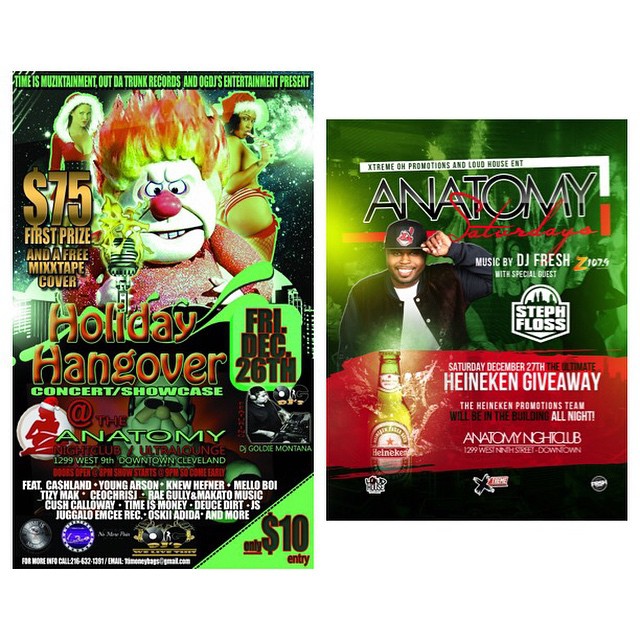Certainly! Here is a cleaned-up and detailed caption for the described image:

---

The composition comprises two adjacent rectangular images. 

**Left Image:**
The left image, resembling a magazine cover, prominently features a clown's face centered in the middle. The clown, with a white face and a bright red nose, has large, expressive white eyes adorned with black dots pointing downward near the nose. Flanking the clown are two women, each slightly tinted green. The woman on the left is dressed in a low-cut red suit accented with a white feathery trim. The woman on the right, donning a Santa Claus hat, is topless, with her arm modestly covering her chest and her rear end pointed towards the clown’s head.

At the top of this image, green text announces: "Monson Cumit, Trunk Records, and Elgast Entertainment present." Adjacent to the clown, a golden text offers a "$75 first prize and free mixtape cover." Further below, the text proclaims: "Holiday Hangover, Friday, December 26th. Concerts Last Schedule: Anatomy." The bottom right corner features a green triangle with the information: "Only $10 Entry."

**Right Image:**
The right image serves as a separate advertisement. A white bar at the top reads: "Extreme Promotions and Loud House." Below this, in black text, is the word "Anatomy." The central figure is a smiling black man wearing a Cleveland Indians baseball cap, his hand lifting the brim. He’s clad in a black open jacket over a white shirt.

Below the man’s portrait, an advertisement showcases a bottle of Heineken on the left side, alongside text on the right: "Saturday, December 27th. Heineken Giveaway." At the bottom, the text reads: "Anatomy Nightclub." The background is filled with various shades of green, ranging from dark hues to lighter shades, especially towards the left side.

---